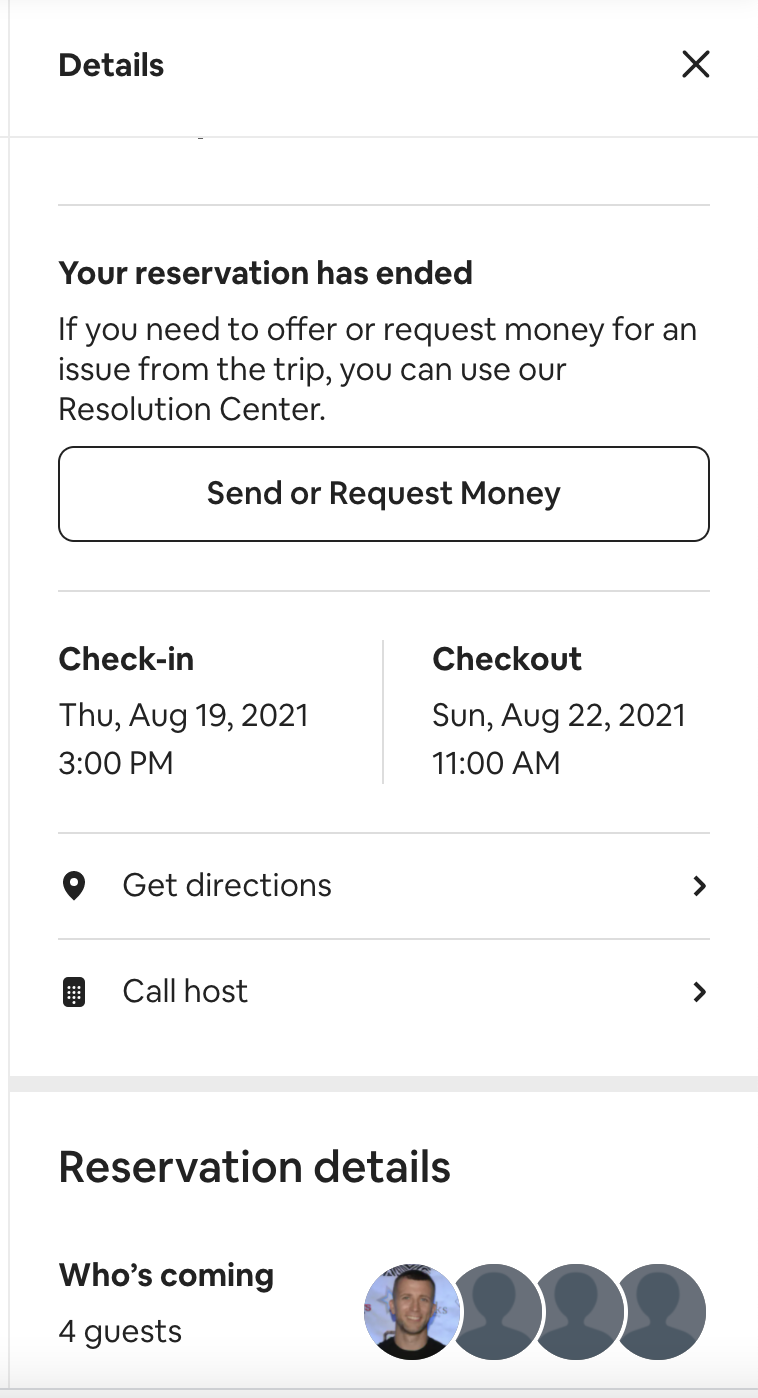Image Description: 

The image depicts a mobile app interface with a white background. The layout is vertical, typical of smartphone screens. At the top left corner, in bold font, the word "Details" is prominently displayed. On the top right corner, there is an 'X' icon intended to close the current view.

A message in the center of the screen reads: "Your reservation has ended. If you need to offer or request money for an issue from the trip, you can use our resolution center." Below this message, there's a white button bordered in black with the text "Send or Request Money" in black font.

Further down, reservation dates are clearly listed in bold: "Check-in: Thursday, August 19th, 2021, 3 PM" and "Check-out: Sunday, August 22nd, 2021, 11 AM." Accompanying these dates are two buttons - "Get Directions" with a GPS icon, and "Call Host" with a phone icon, suggesting additional options available upon clicking.

The section labeled "Reservation Details" follows, summarizing the guest information. It notes "Who's Coming: 4 guests," and includes a profile image of a young man in a black shirt, smiling. Alongside this image are three gray profile icons, likely representing the additional guests.

The overall design of the interface is clean and user-friendly, designed to provide essential information about the booking in a straightforward manner.